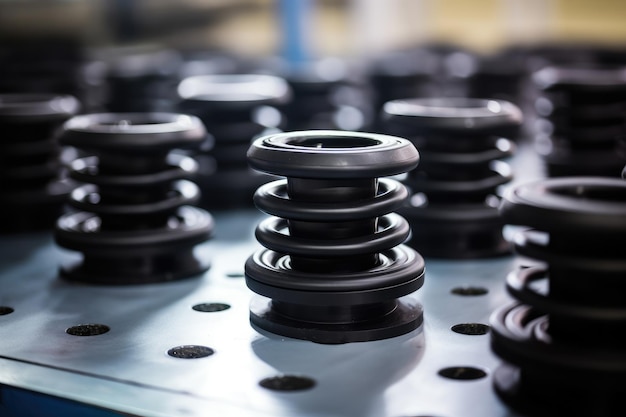This close-up photograph captures a series of mechanical components arranged on a brushed stainless steel surface. The components, possibly machine parts, are composed of black plastic. Each part features a flat base and several concentric rings stacked vertically, creating a spring-like appearance. Interspersed among these intricate black plastic pieces are small, flat black discs that lay directly on the stainless steel surface, adding to the industrial aesthetic of the image.